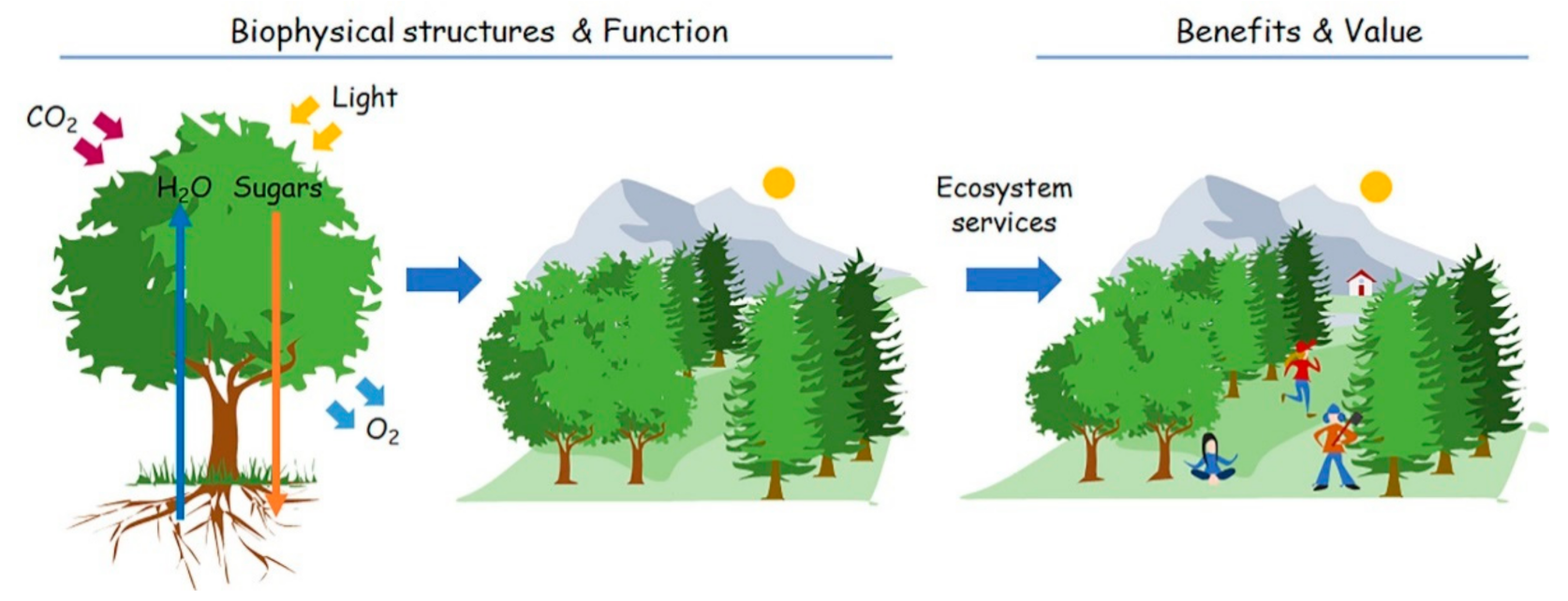The image is a detailed illustration, possibly from a science book, showcasing the biophysical structures and functions of trees, as well as their benefits and values. On the left, the biophysical interactions are highlighted: CO2 from the atmosphere and light from the sky are absorbed by the tree, while H2O is taken up through the roots. The tree produces sugars and releases O2 through its leaves, which supports various ecosystem services. Adjacent to this depiction, a cross-sectional view of the tree's roots and interactions is shown, leading to a broader scene of a thriving ecosystem. In the subsequent visuals, a grouping of trees is seen with a background of mountains, a house, and people engaging with nature—jogging, doing yoga, and even someone carrying an axe. These activities illustrate the diverse benefits and values of forests, including clean oxygen, recreational spaces, and the presence of a healthy ecosystem.